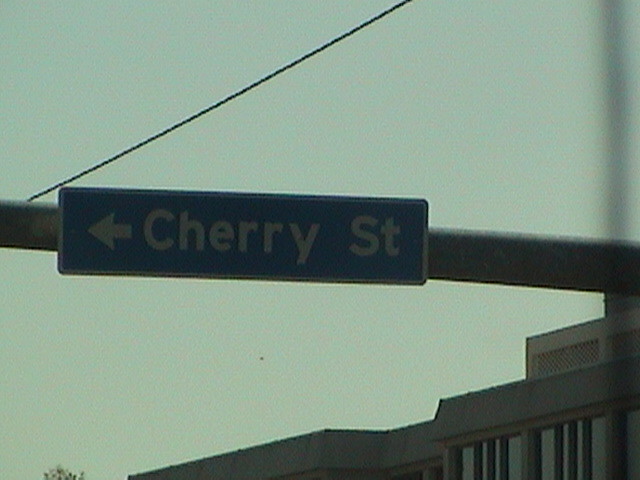This photograph features a dark green, rectangular street sign with "Cherry Street" written in bold white letters and an arrow pointing left. The sign is suspended from a metal pole, possibly part of a traffic light structure. A black metallic cable runs diagonally from the lower left corner to the upper right center of the sign. In the background, a large gray building, likely an office building or courthouse, is visible. The sky is overcast, exhibiting shades of light blue and green. The image appears to be taken from inside a vehicle or just outside on the street.